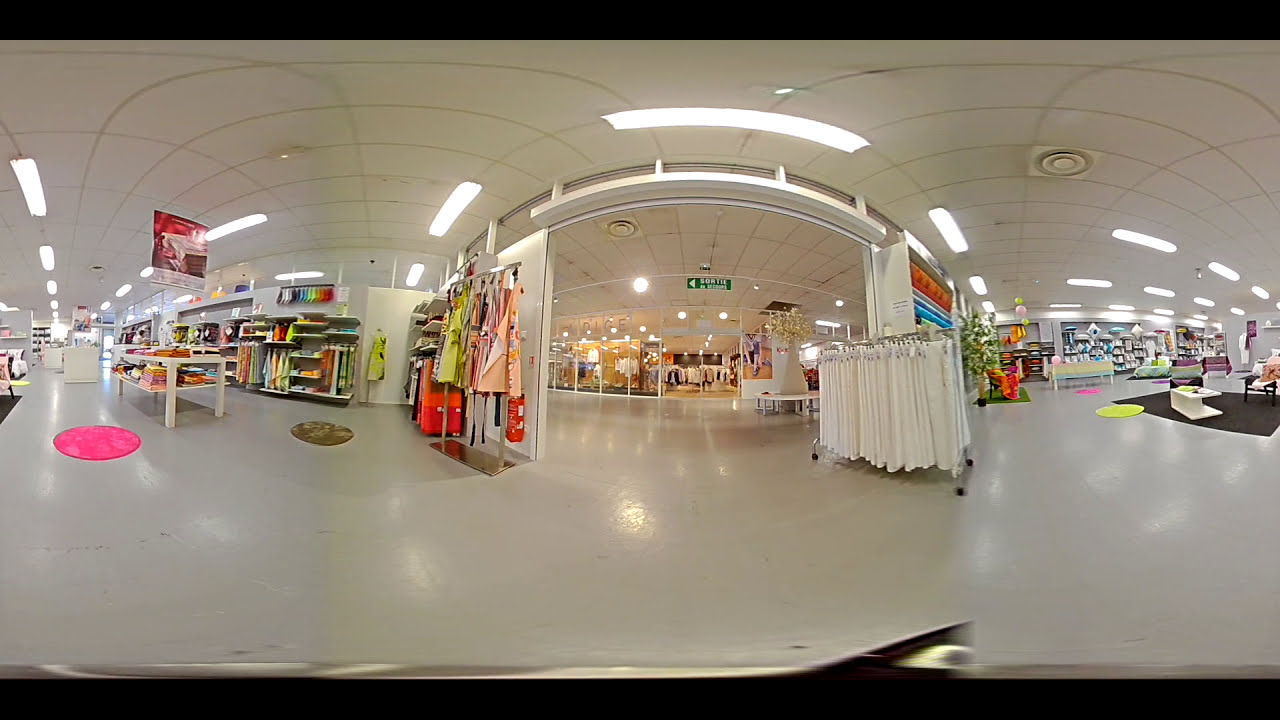The image captures a somewhat low-resolution, wide-angle security camera or surveillance footage of a large department store with tiled, glossy white floors that reflect the overhead fluorescent lighting set into panel ceilings. The store is well-organized, with various sections and items on display. Prominently, the camera is positioned to face the store’s entrance, which reveals another store directly across.

On the left side of the image, the store features multiple shelves along the wall displaying an assortment of colorful clothes and items, including orange, pink, and yellow garments hanging on freestanding clothes racks. There are also several tables stacked with neatly folded clothing. Distinct circular patterns in pink and light brown can be seen on the floor.

In the center of the image, we see the main entrance leading into an open space marked by a green sign hanging from the ceiling. Right inside the entrance is a moving clothing rack filled with white pants. Opposite the entrance, there's a seating area with a circular bench and glass windows showcasing more clothing racks.

To the right side of the store, the image captures additional seating arrangements with cushions, small tables, and more shelves running along the wall. This area appears to blend into a section possibly dedicated to home furnishings, including beds and bedding, contrasting with the primarily clothing-focused setup on the left side of the store. Overall, the scene conveys a busy, well-lit retail environment designed to cater to a variety of shopping needs.